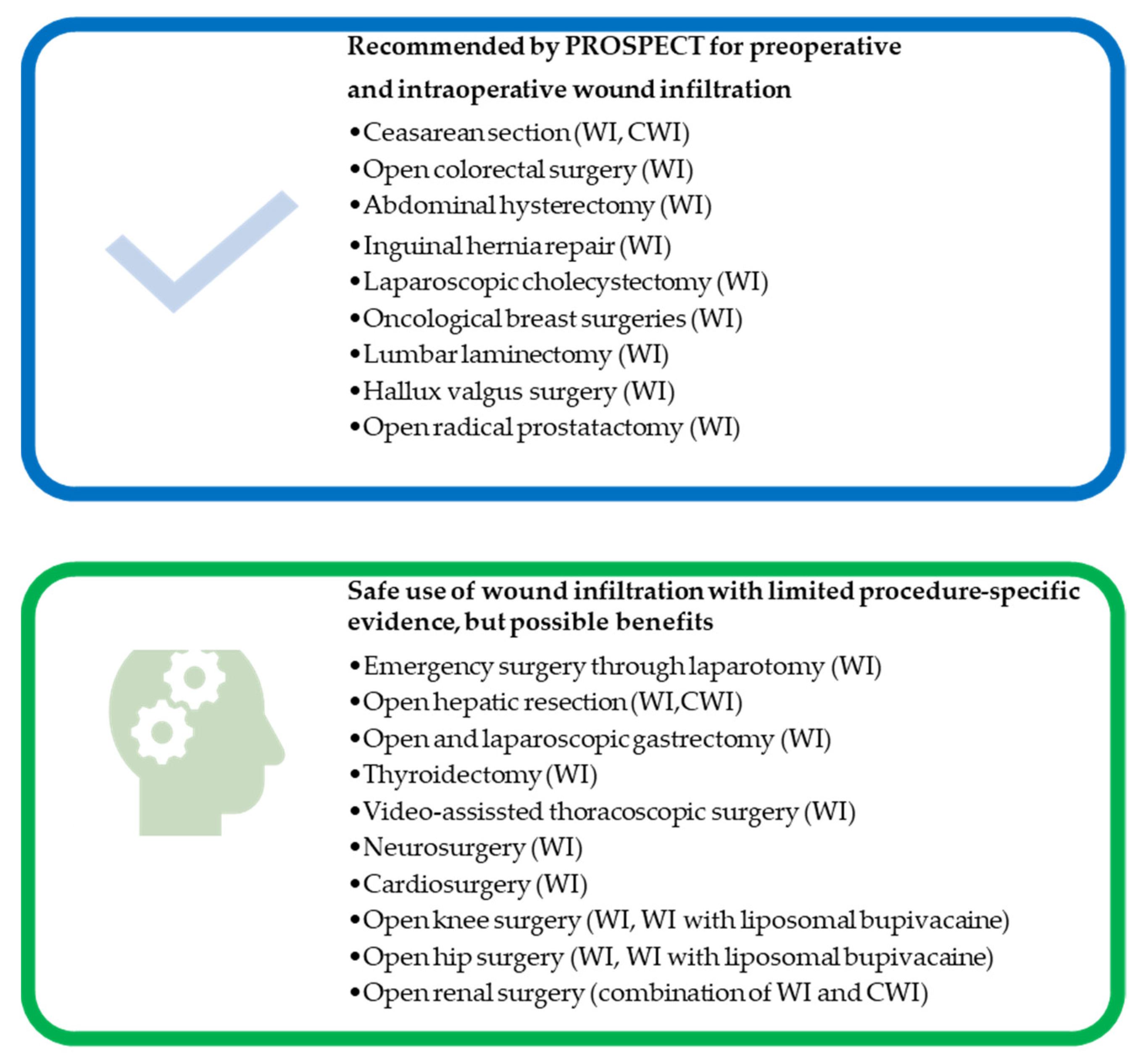The image is an informational poster comprised of two main outlined sections. The top section is encased in a blue rectangle with a light blue check mark on the left side. It is labeled "Recommended by Prospect for Preoperative and Intraoperative Wound Infiltration" and lists specific surgical procedures such as open colorectal surgery, abdominal hysterectomy, inguinal hernia repair, laparoscopic cholecystectomy, oncological breast surgeries, lumbar laminectomy, hallux valgus surgery, and open radical prostatectomy. The bottom section, outlined in green, features a profile illustration of a green head with two white gears inside. It is titled "Safe Use of Wound Infiltration with Limited Procedure Specific Evidence but Possible Benefits" with several bullet points elaborating on the benefits. The layout is visually segmented to clearly distinguish between the recommendations and evidence-backed safe practices for wound infiltration in surgical procedures.